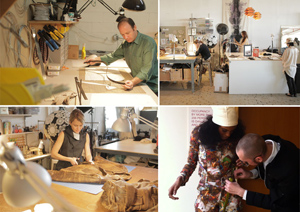The image is a collage of four distinct photographs arranged in a grid, each depicting individuals engaged in various activities. In the upper left corner, a man wearing a green long-sleeve shirt sits at a desk under the focused light of a v-shaped desk lamp, sketching on paper amidst a workbench filled with tools. Adjacent to this scene, the upper right corner features a somewhat distant image of a factory setting where several individuals are gathered around a work table with a white cover. Below this, in the lower left corner, a woman dressed in a black short-sleeved outfit, with her hair pulled back, diligently cuts cloth on another work surface. Finally, the lower right corner depicts a black woman in a floral outfit with a white hat standing next to a white man in a suit, who appears to be adjusting something around her waist or stomach.